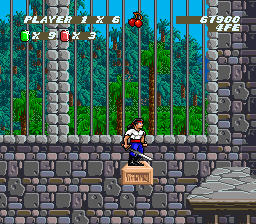The image is a still from a computer or video game showcasing a detailed scene. The background features a stone wall composed of an assortment of stones and bricks in various sizes and colors, including smaller pink and blue stones alongside larger gray square stones, and horizontally longer olive green and gray bricks. In front of the wall, silver-gray bars resembling those of a jail cell rise, hinting at some form of confinement.

Behind the bars, a lush, vibrant landscape unfolds, with a mix of tropical palm trees and evergreen trees, their trunks extending upwards toward a bright blue sky. Amid this scene, the focal point is a character standing on a wooden block against the stone wall. This character is striking and detailed, dressed in blue pants, black boots, a red belt, and a white muscle shirt that shows off his physique. He sports a red headband or bandana around his head, has black hair pulled back into a ponytail, and holds a metal sword with a silver blade and a brown handle in his right hand.

Overlayed onto this intricate background are game elements including a scoreboard with "PLAYER ONE x6" and an F for FE marking beneath it. Also visible are items like a set of red cherries, a green gem, and a red gem, along with indicators "X9" and "X3," adding to the immersive gaming experience.